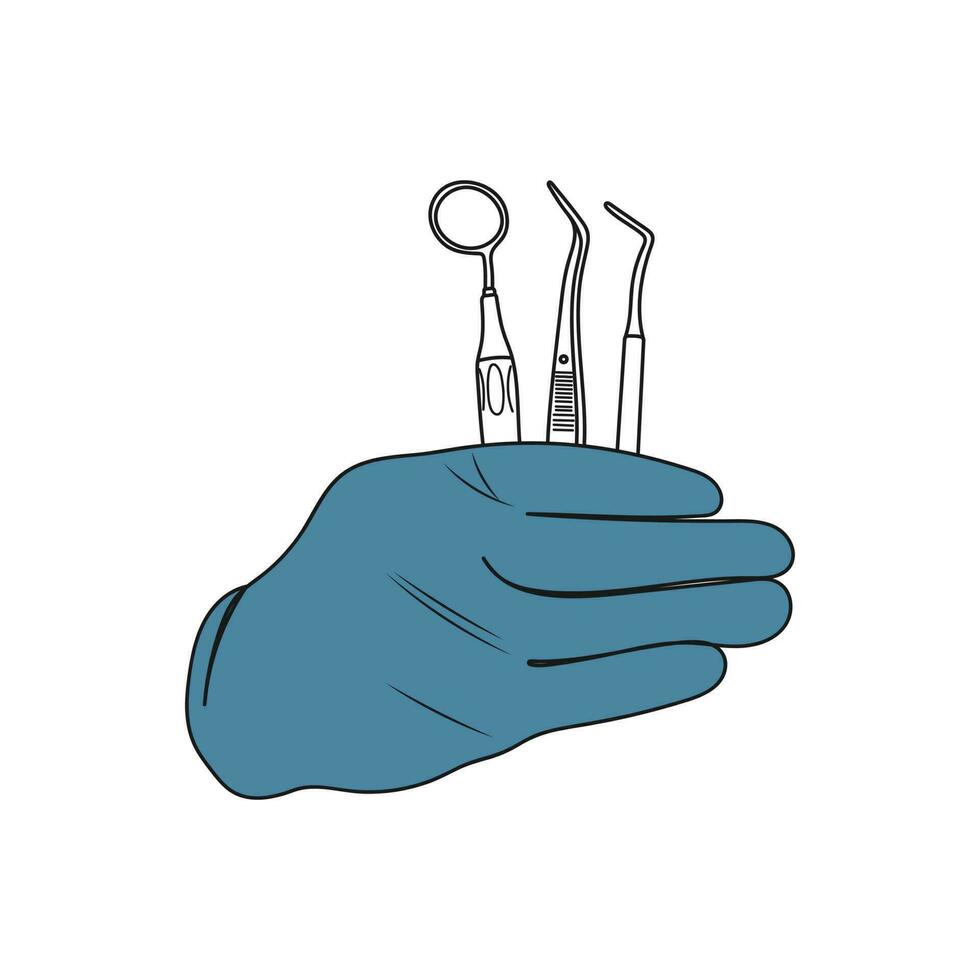This is a detailed digital rendering of a hand wearing a turquoise, almost dark teal latex glove, holding three dental instruments against a completely white background. The image has a minimalist, textbook-like quality, with the hand and instruments outlined as if drawn digitally. You see the four fingers from the back, with the thumb obscured around the side. The glove shows slight wrinkles where the fingers bend, adding to the realistic feel.

The dental instruments consist of a small mirror on a stick to the left, likely used for inspecting within the mouth, and two dental picks with bent ends for scraping and pulling tartar. The leftmost instrument has a long handle featuring an oval-patterned grip and a circular end. The middle pick has a grooved handle, designed for a firm grip, with a single bend at the top to the left, ending in a sharp point. The rightmost pick has a straight, ungrooved handle with a similar single bend at the top to the left.

Overall, the simplicity and precision of the image, with its focus on the gloved hand and the dental instruments against a stark white background, give it a clinical, scientific appearance, reminiscent of an illustration you might find in a medical textbook.